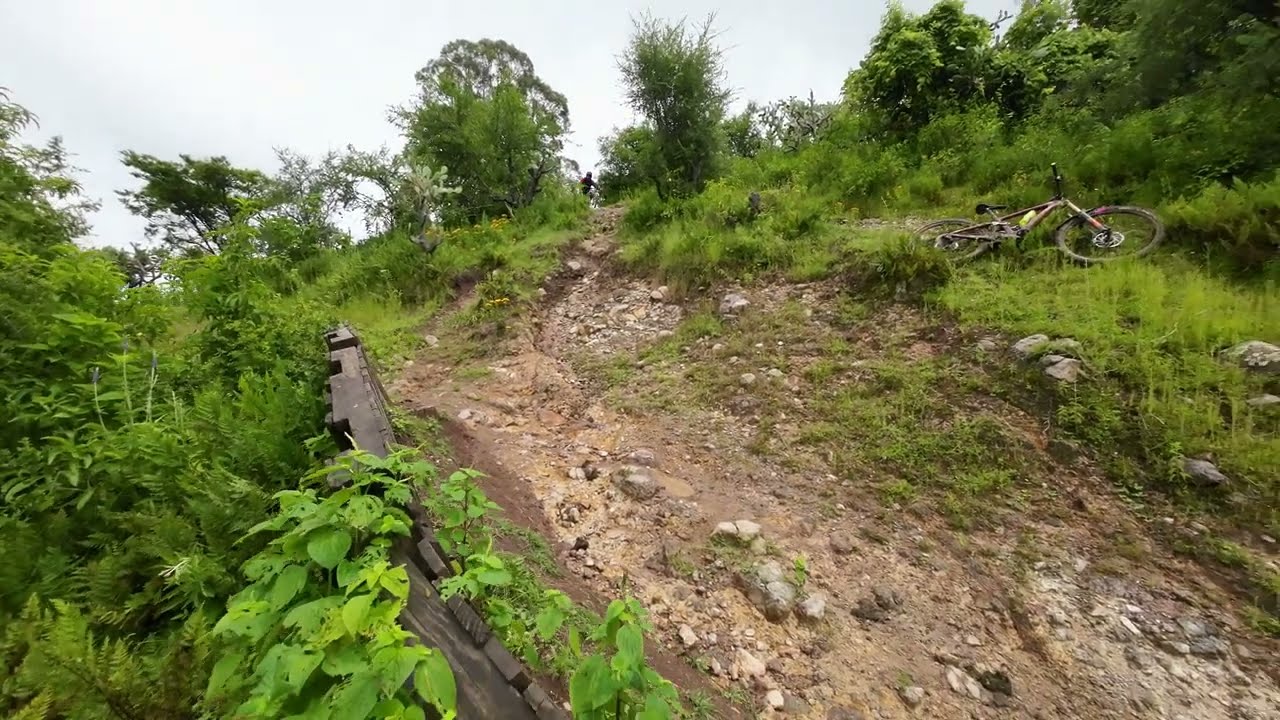The image features a rugged mountain bike trail characterized by its beige and brown dirt mixed with white rocks and gravel. The trail is bordered by a small, three-foot tall dark grey wooden fence, with lush greenery on the left side. On the right side of the fence, the trail sprawls with speckles of green foliage around it, and there's a lot of moss and overgrown plants, indicating it's not well maintained. Towards the upper right of the image, a lime green water bottle can be seen strapped to a mountain bike lying on its side, partially obscured by the grass. Further up the trail, a distant figure wearing all black can be seen either pushing or riding a bike toward the foreground. The backdrop fades into an overcast sky, creating a gray tone over the scene. On the horizon line, trees frame the top of the hill, adding to the rugged and natural ambiance of the landscape.